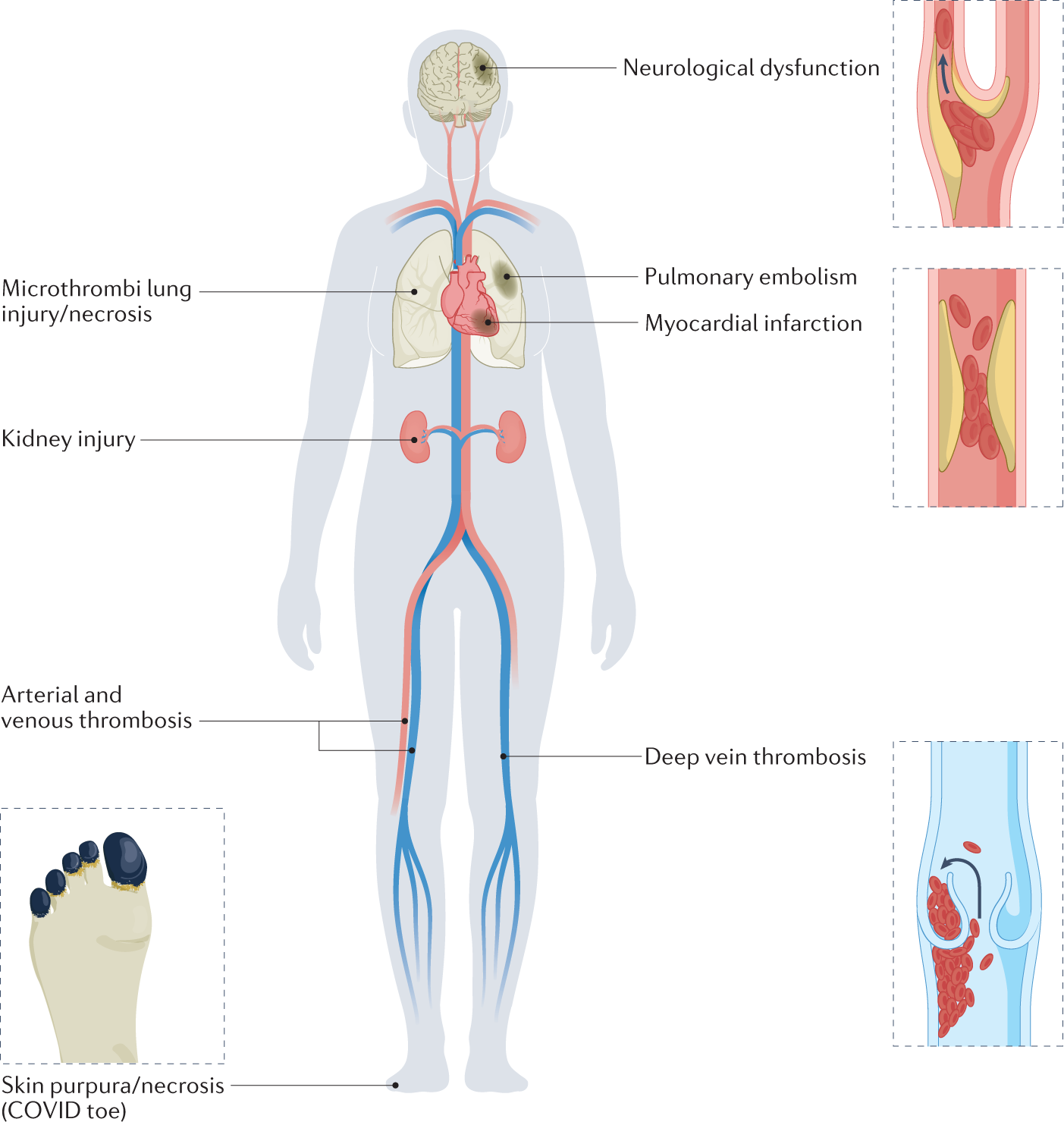This detailed image, likely from a biology textbook, illustrates various medical conditions affecting different organs within the human body. The central figure is a grayish, transparent outline of a human body, revealing internal organs such as the brain, lungs, heart, kidneys, and major arteries. Specific sections are highlighted and expanded upon with text and detailed diagrams. For example, the brain is labeled with "neurological dysfunction," pointing at the left side of the brain. The lungs are marked with "pulmonary embolism" and "microthrombi lung injury necrosis." The heart is labeled "myocardial infarction," with a detailed view on the right showing an artery, illustrating how high-density lipoproteins obstruct blood flow, leading to clots and heart attacks. The diagram also highlights "kidney injury," "arterial venous thrombosis" in the veins towards the knee, "deep vein thrombosis" at the knee, and "skin purpura necrosis" indicated as COVID-toe.